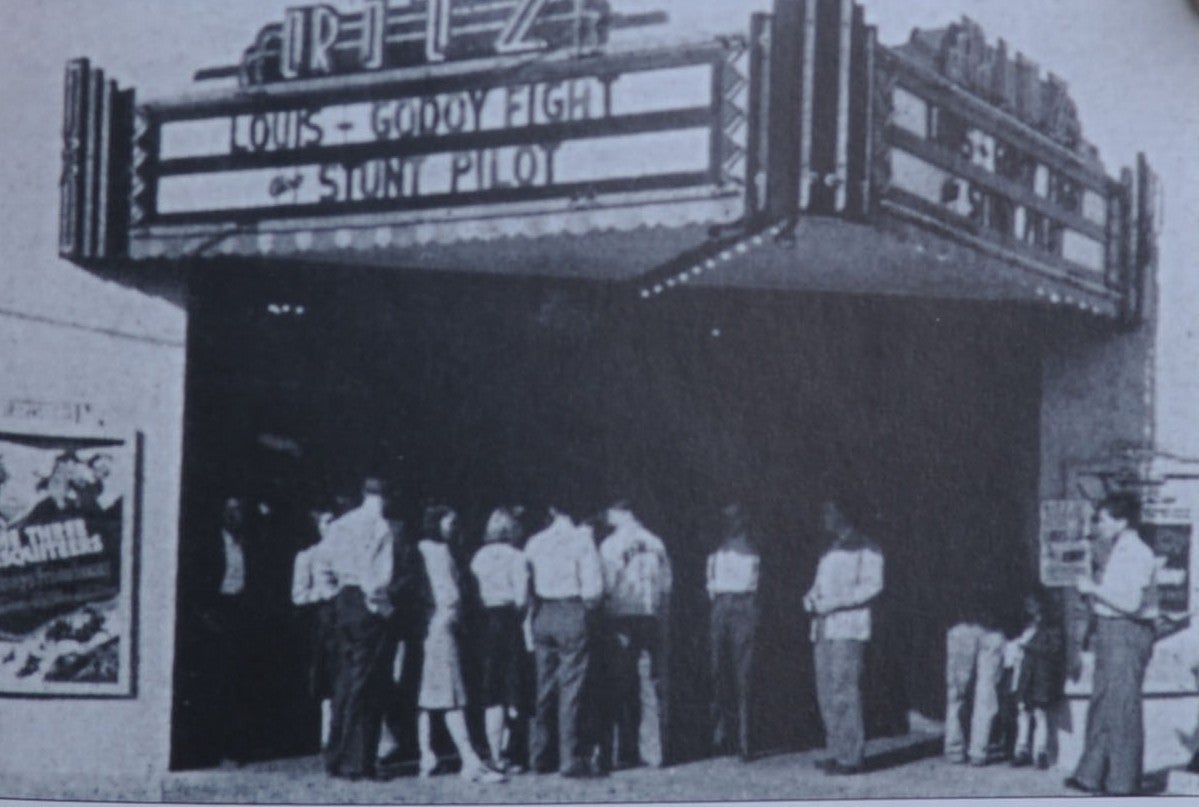The image is a very old, black-and-white photograph depicting the exterior of a vintage movie theater, likely from a retro era. The theater has a traditional façade, featuring a prominent triangular overhang with neon letters that spell "Ritz" above it. On either side of the overhang, there's text that reads "Louie Goodboy Fight" on the first line and "Stunt Pilot" below it in bold black on white lettering. Despite the photograph being blurry and pixelated, and somewhat underexposed, several people, around 15-20, can be seen standing in a queue outside the theater. The shadowy area underneath the overhang obscures detailed visibility, but those outside the shadow are clearly illuminated by sunlight. The individuals appear to be dressed in period-appropriate attire, with men in shorts and pants, and women in long skirts. Posters are also visible on the left and bottom right walls, adding to the classic theater ambiance.